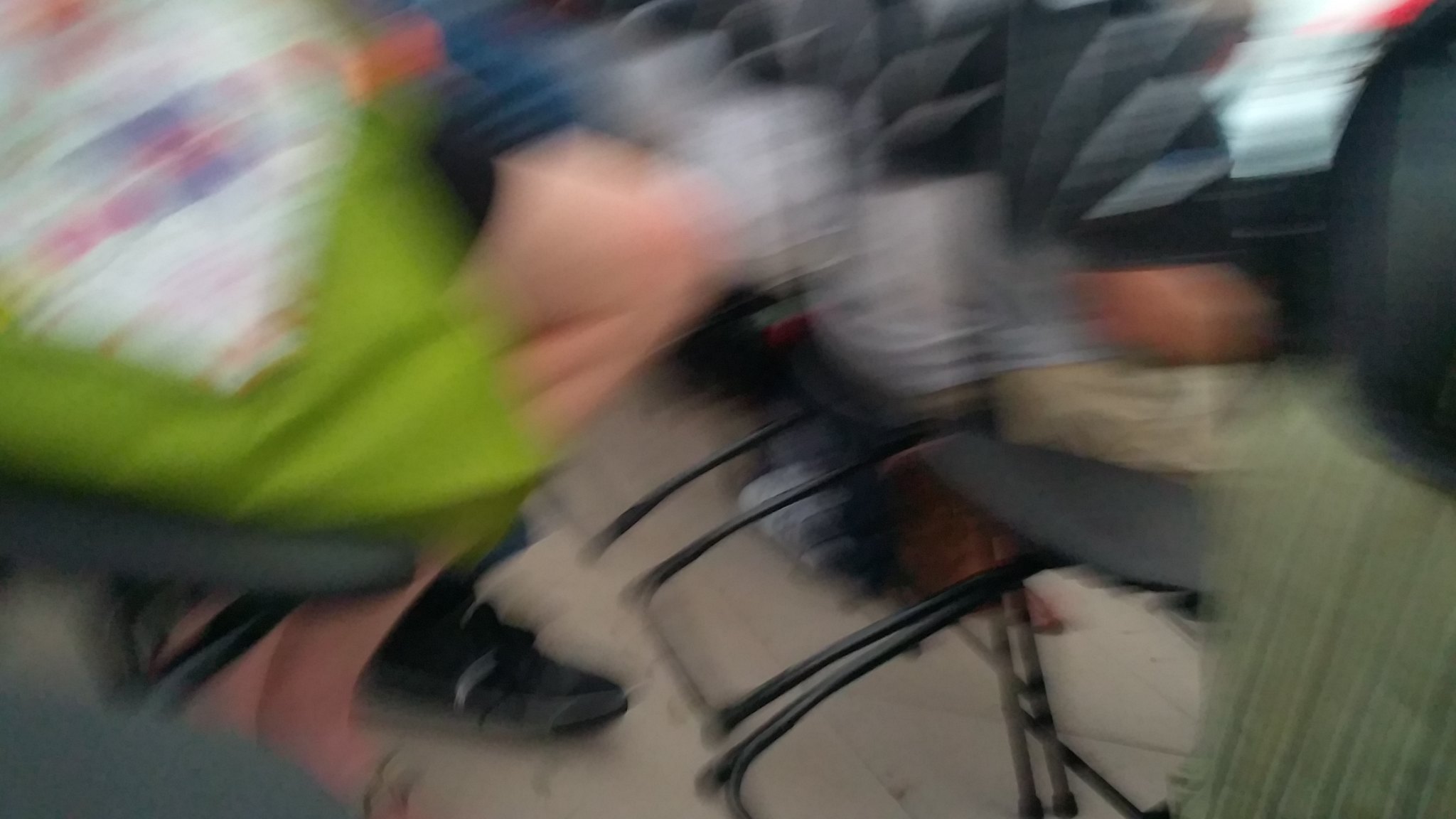A motion-blurred photograph capturing a scene of several people seated on simple stools, characterized by round black seats supported by metal frames. Due to the significant motion blur, the details of the image are somewhat obscured, making it challenging to discern clearly. One identifiable figure is a man in green shorts, whose white leg extending from the shorts is visible, along with his black shoes. In the foreground, a woman in a green dress is discernible; her tanned arm is exposed and she is wearing a white shirt. The overall sense of movement suggests the photo was taken while the camera or the photographer was in motion.